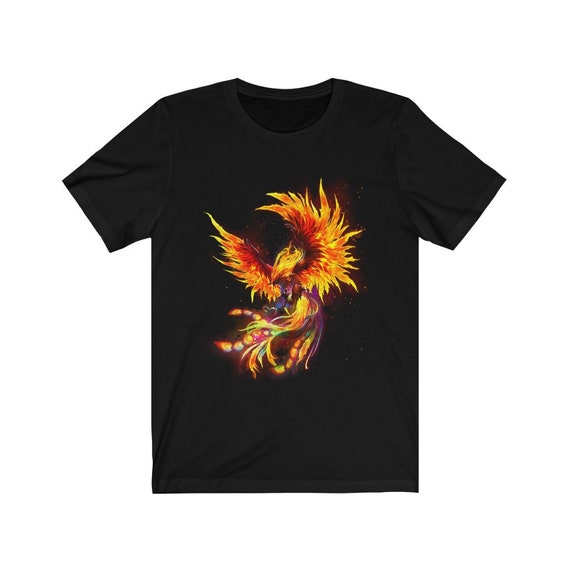The image features a centrally positioned black medium-sized t-shirt with short sleeves and a round neckline, set against a plain white background. The centerpiece of the t-shirt is a vivid graphic illustration of a phoenix-like creature. This mythical being has striking, angel-like wings that appear to be ablaze with vibrant shades of orange and red, giving the impression of fire. The creature possesses a glowing yellow head and a mesmerizing purple tail that blends with hues of orange, yellow, and blue, accented by shades of green. The intricate design adds an abstract, almost fantastical element to the shirt, making it a standout fashion piece.